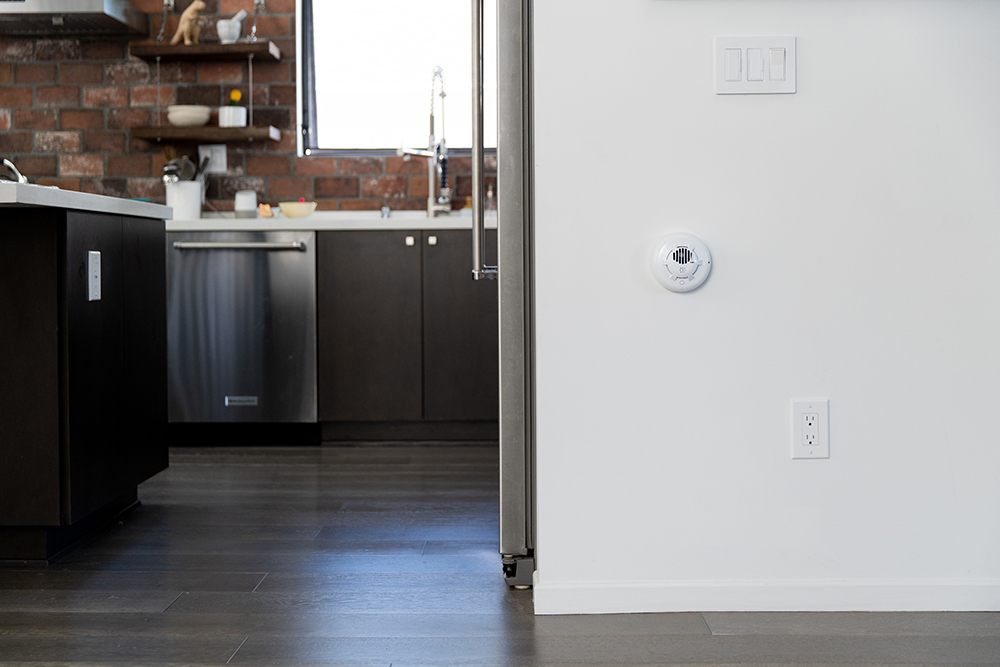This detailed photograph captures a stylish kitchen from an entryway perspective, blending the kitchen and hallway elements. The kitchen cabinets are predominantly dark brown or dark grey, contrasted by white countertops. Stainless steel appliances, including a visible dishwasher and refrigerator handle, add a sleek touch. The back wall features brick-shaped brown tiles and is adorned with freestanding wood shelves holding white pottery. In the center, a sink with a silver faucet sits below a window, through which glaring light pours in. To the right, a white wall displays three light switches, a circular vent, and a three-pronged outlet. The floor is dark gray wood, extending to an island with a dark cabinet base and a white countertop, exemplifying modern interior decoration.